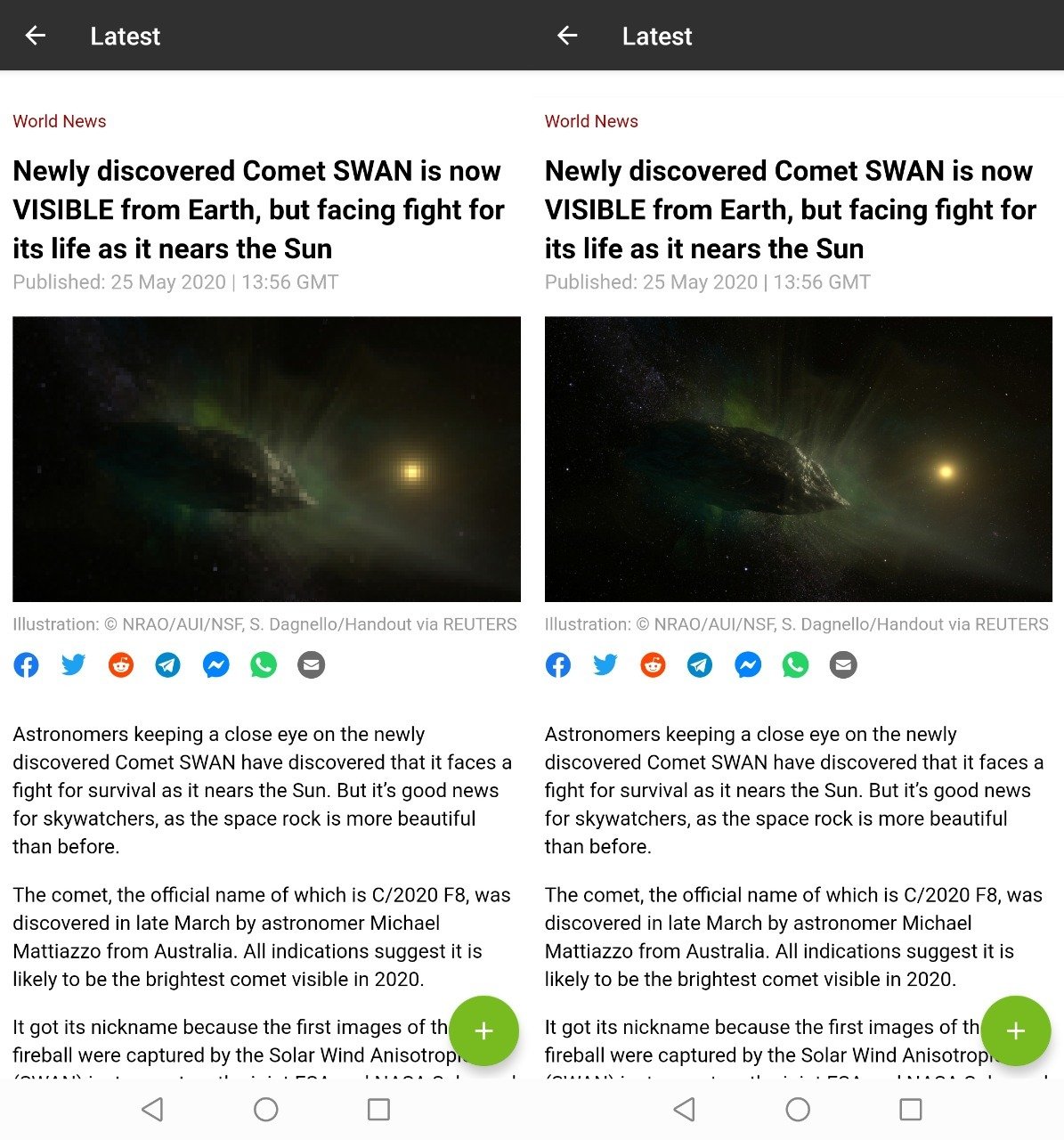The image features two nearly identical articles side-by-side, each with a black banner running across the top. On both banners, there's an arrow pointing left next to the word "Latest" in bold text. This layout is mirrored on the right side. Below the banner, a section marked "World News" appears in burgundy red, followed by the article's title in bold black text: "NEWLY DISCOVERED COMET SWAN IS NOW VISIBLE FROM EARTH FACING FIGHT FOR ITS LIFE AS IT NEAREST THE SUN."

The article is dated May 25th, 2020, at 13:56 GMT. Both articles include an image of Comet SWAN, but the image on the left is noticeably blurry, while the image on the right is crisp and clear. The comet is depicted with a greenish hue, and there's a slight yellow light visible on the center-right side of the comet in both images.

Beneath each image, there's a segment of the article providing more details about the comet. A green circle with a plus button is prominently featured below the images, offering options to share through multiple platforms, including Facebook, Twitter, Reddit, Telegram, and Messenger.